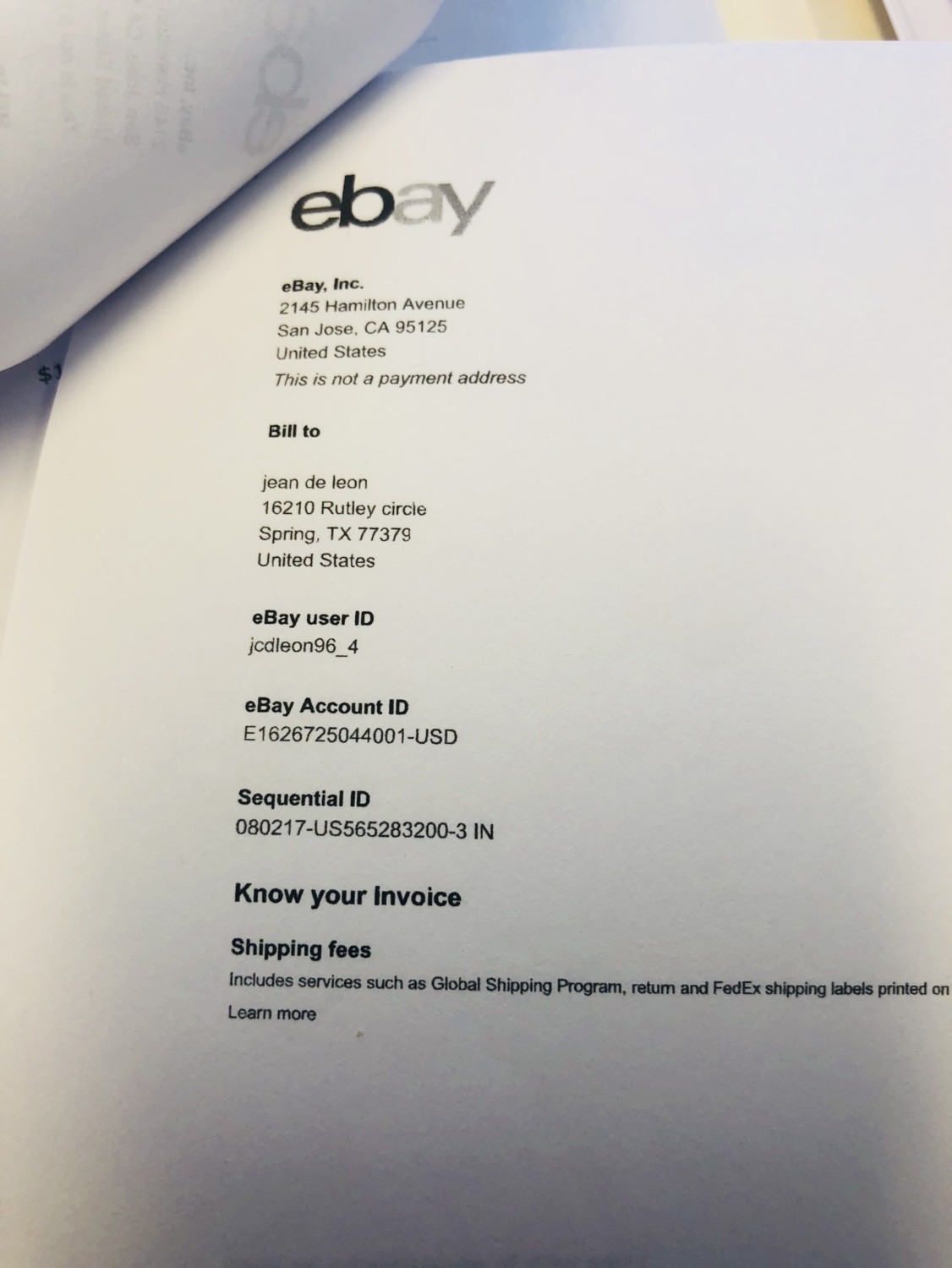The image depicts a detailed eBay invoice printed on a white sheet of paper with black lettering. At the top of the page, "eBay" is prominently featured in large, stylistically varying shades of grey, with "EB" notably darker than "AY." Below the logo, the address for eBay Incorporated—21543 Hamilton Avenue, San Jose, California 95125, United States—is listed, with a clarification that it is not a payment address. The "Bill To" section lists Jean de Leon at 16210 Rutley Circle, Spring, Texas 77379, United States. Following that, specific details for the eBay user—in this case, the username "Jcdleon96"—are provided along with the eBay Account ID: "e16262055044001-USD" and Sequential ID: "080217-US565283200-3."

Towards the bottom of the document, in bold black letters, it says "Know Your Invoice," and it explains that shipping fees include services such as the Global Shipping Program, Return, and FedEx Shipping Labels, followed by a prompt to "Learn more." The appearance of additional pages staples together and flipped off to the top left corner indicates that this invoice is part of a multi-page document, although the details on the other pages are not visible.